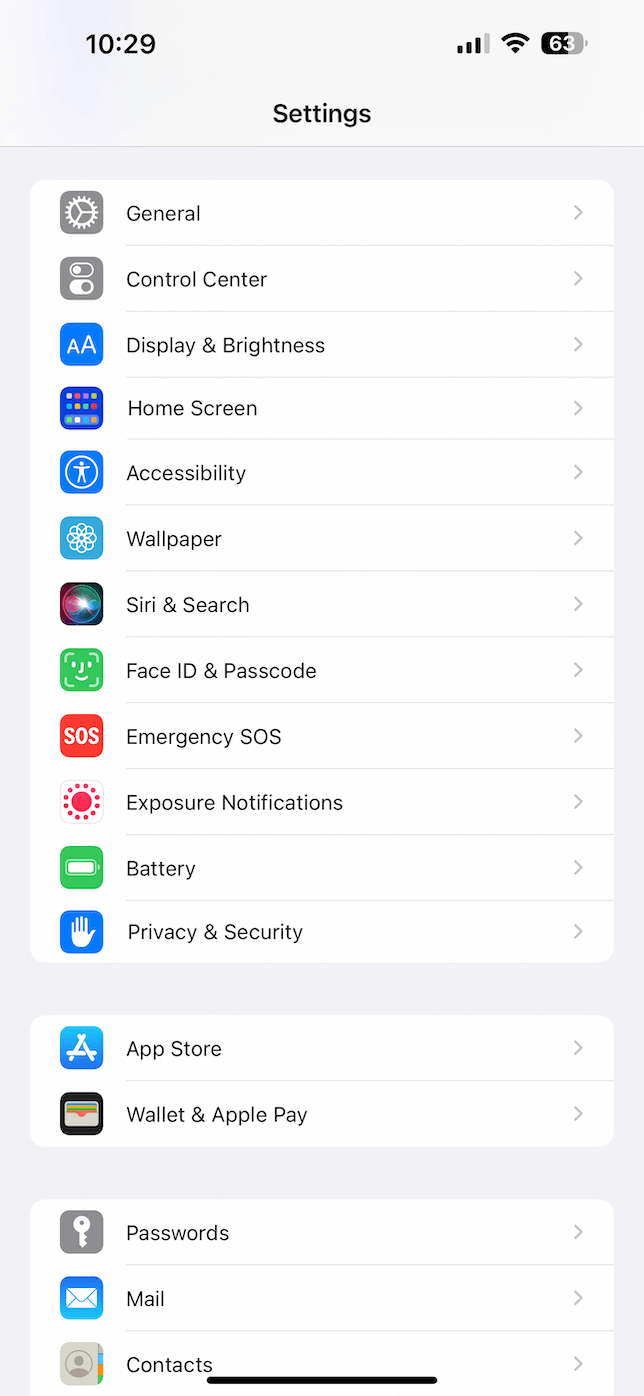The image depicts a screenshot of someone's iPhone home screen, featuring the "Settings" menu interface. The top part of the screen shows a typical status bar with several indicators. In the upper left corner, there is the current time displayed as "10:29." The status bar also shows three filled service bars, indicating decent cellular reception. Next to it, the Wi-Fi icon is filled, signaling a strong Wi-Fi connection. The battery percentage is displayed as "63%", and there is a moon icon indicating that the 'Do Not Disturb' mode is activated.

Below the status bar, the screen lists several settings options divided by thin gray lines. Each section starts with a rectangular label. The categories listed, in order, are:

1. **General** - A line separating.
2. **Control Center** - Another line separating.
3. **Display & Brightness** - Another line separating.
4. **Home Screen** - Another line separating.
5. **Accessibility** - Another line separating.
6. **Wallpaper** - Another line separating.
7. **Siri & Search** - Another line separating.
8. **Face ID & Passcode** - Another line separating.
9. **Emergency SOS** - Another line separating.
10. **Exposure Notifications** - Another line separating.
11. **Battery** - Another line separating.
12. **Privacy & Security** - Another line separating.

Towards the bottom, there is another rectangular section featuring:

1. **App Store** - A line separating.
2. **Wallet & Apple Pay** - Another line separating.
3. **Passwords** - A line separating.
4. **Mail** - A line separating.
5. **Contacts** - Completing the list.

The overall screenshot provides a clear view of various settings options available on the device, with the clean and systematic display typical of iPhone interfaces.